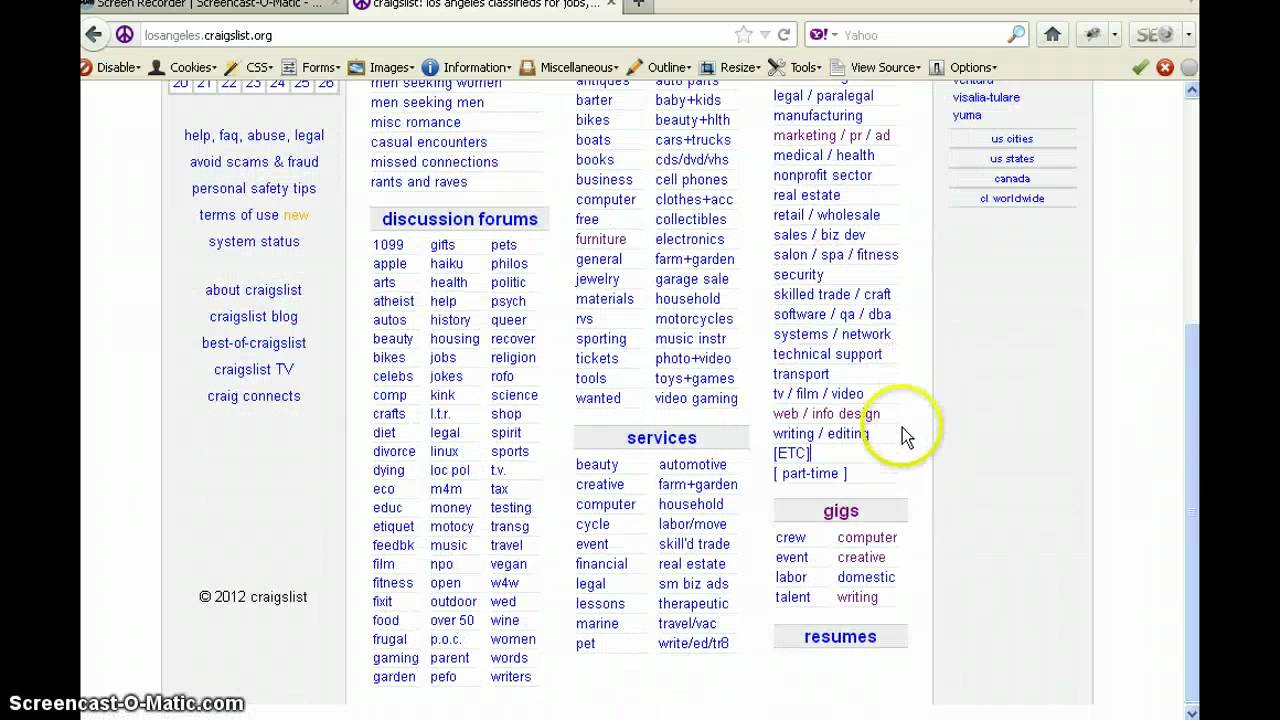This image captures a detailed view of a Craigslist webpage. Prominently featured is a search bar at the top, within which an inquiry about Los Angeles has been partially typed, though the text appears skewed and indistinct. The familiar sparse design of Craigslist is evident, characterized by its extensive list of categorized sections available for browsing. These sections include discussion forums, various services, and an array of items for sale like furniture, general merchandise, jewelry, and computers.

On the left-hand side, a vertical box is clearly visible, containing links to essential resources such as "help," "frequently asked questions," "abuse/legal," and "avoid scams and fraud." This box provides users with crucial assistance and safety information. Below these links, the site offers additional support and insights into Craigslist through sections labeled "Craigslist blog," "best of Craigslist," "Craigslist TV," and "Craig Connects."

Above these sections, the site navigation includes options like "images," "information," "outline," and "view source," providing various viewing and information-gathering capabilities. On the right-hand side of the page, there are links categorized under "Yama," which encompasses a directory of cities, states, Canada, and worldwide locations, enabling users to find pertinent listings or resources in specific geographic areas. This comprehensive layout is designed to aid both new and experienced users in navigating the multifaceted platform of Craigslist.